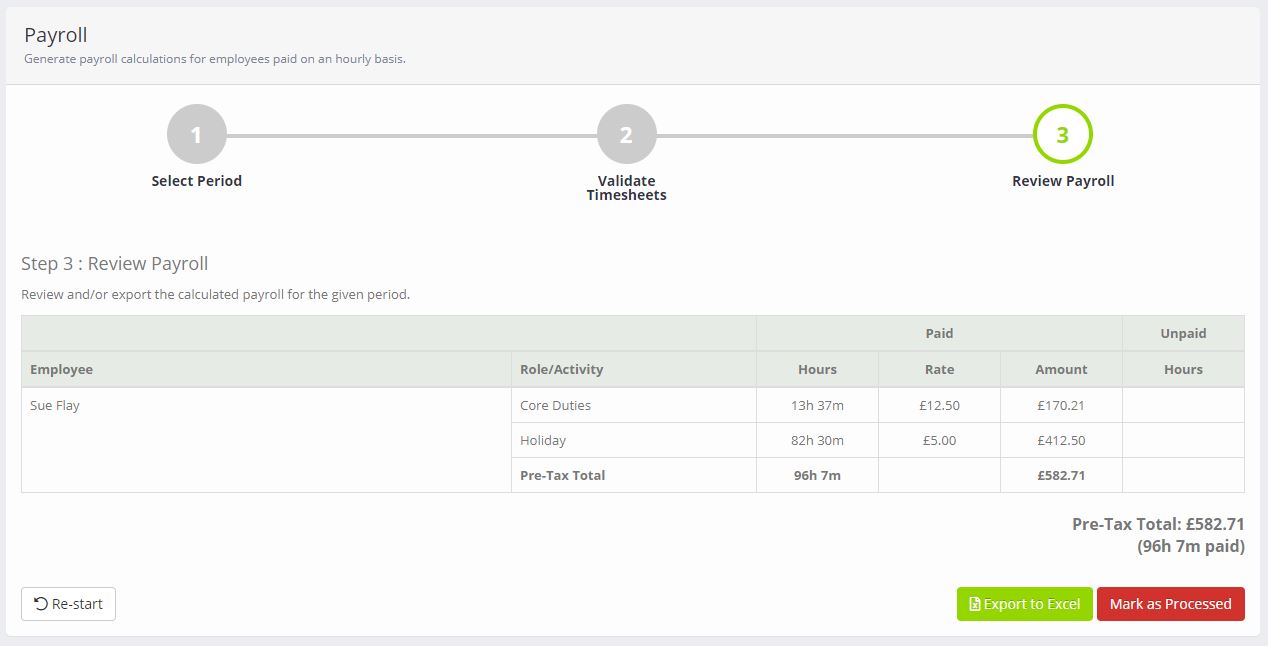This is a detailed screenshot of a payroll application interface designed for employers and payroll administrators. The screen is titled "Payroll Generate" and focuses on payroll calculations for employees paid on an hourly basis. 

At the top, a process flow is illustrated with a line graph indicating three key steps:
1. Select Period
2. Validate Timesheets
3. Review Payroll.

Currently, the application is in step three, "Review Payroll," where users can review and/or export the calculated payroll data for the selected period.

Below this process flow, there is a detailed chart titled "Employee Souffle Role Activity." This chart breaks down various components of the employee’s payroll hours and activities:
- Core Duties: 13 hours, 37 minutes
- Holiday: 82 hours, 30 minutes
- Pre-tax Total: 95 hours, 7 minutes 

The employee's pay rates are as follows:
- Regular hours at €12.50 per hour
- Holiday hours at $5.00 per hour

The total earnings for this period include:
- €170.21 for time worked
- €532.71 as the combined total with all components included

At the bottom right corner of the screen, there are two buttons, one red and one green, presumably for approving or rejecting the payroll data.

This well-organized interface provides a comprehensive overview and facilitates accurate payroll management.